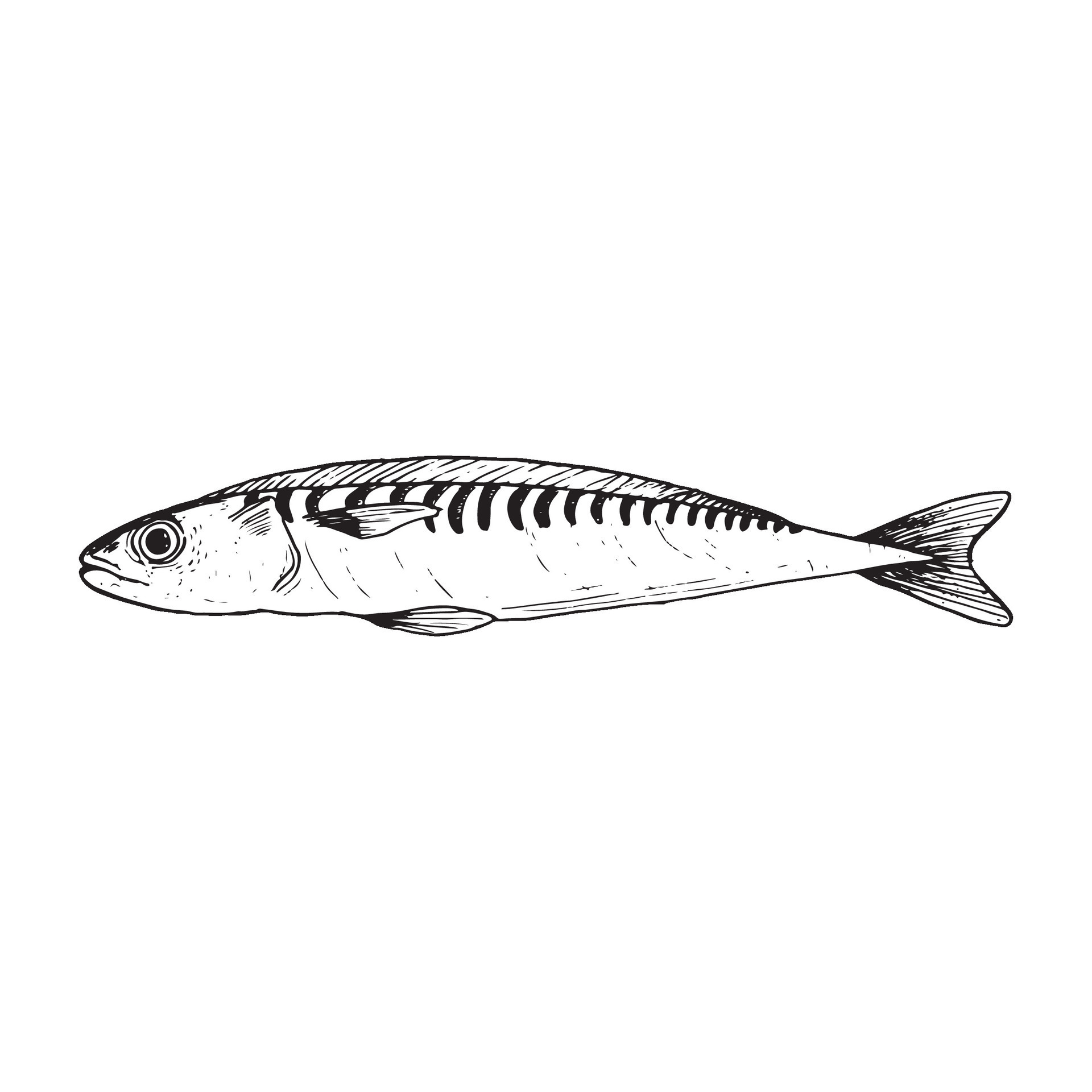This black and white illustration features a slender, long fish set against a pure white background. The fish occupies nearly the entire horizontal space of the image, facing left with a flat, rounded head and a slightly open mouth. It has a prominent large eye with a white outline and a large black pupil. The body of the fish is quite thin, tapering to a sharp point on the right where the tail emerges. The tail, shaped like a boomerang, curves gently downward. The fish is adorned with a series of black stripes along its top, which extend about a third of the way down its body. There are three visible fins: a long arcing fin on top with angled black lines, a pointy fin near the top, and an elliptical fin on the bottom with horizontal black stripes.